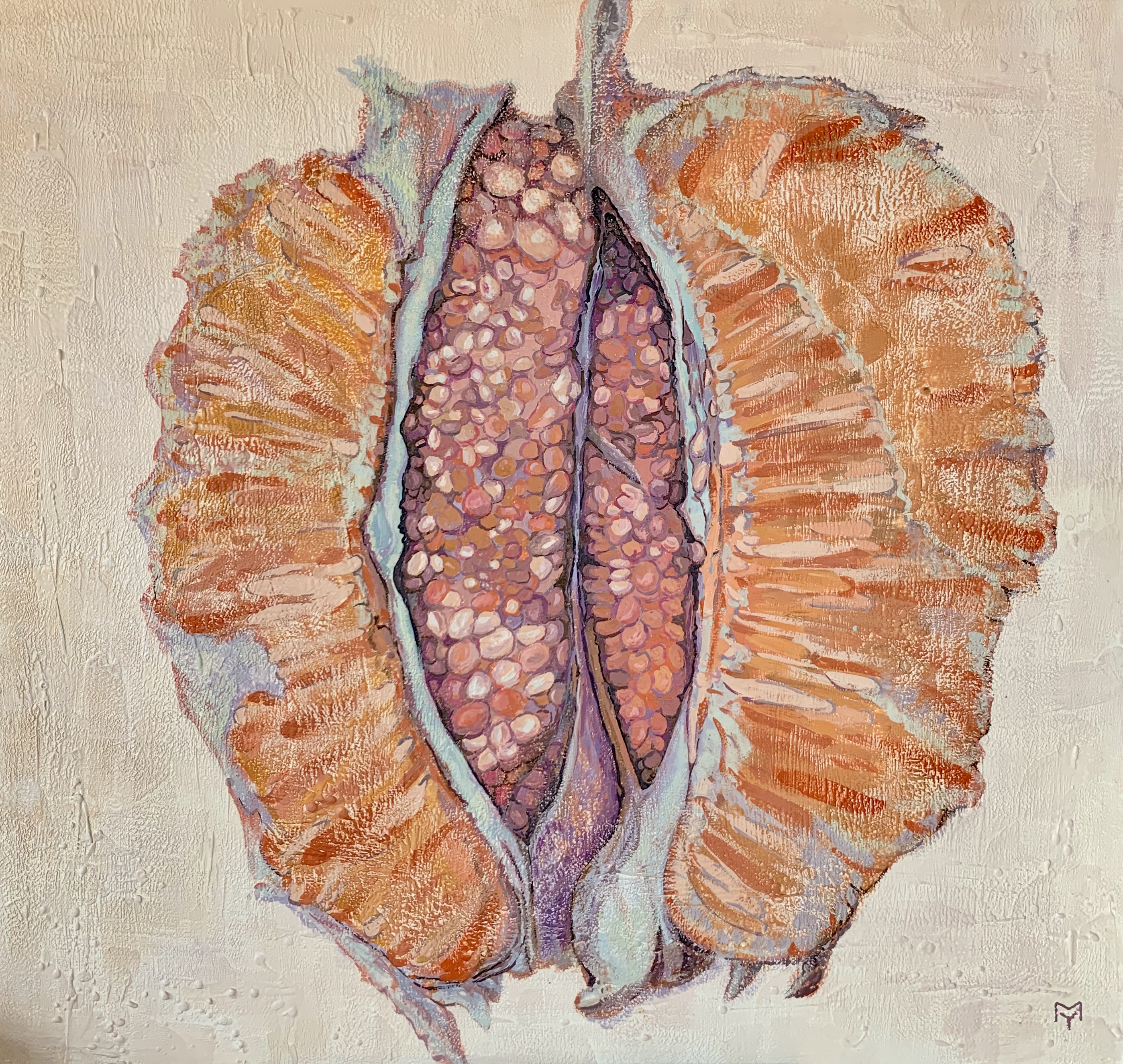The image is a detailed illustration, likely a painting or drawing, of what resembles the inside of a dried-up and slightly shriveled fruit, possibly an orange. The background of the artwork features a light cream or tan color with darker areas that give it a grunge or weathered texture. The outer edges of the fruit are shades of orange, varying from deep to lighter hues, with a slightly shriveled appearance, giving it a realistic, aged look. This orange border encloses two large sections that prominently display the characteristic fleshy texture and white veins typical of an orange's interior. 

In the center of these sections, there is an intricate design featuring white spines or arcs surrounding numerous small brown and white seeds, reminiscent of a pomegranate's interior. These seeds are densely packed, contributing to a complex, almost beaded texture with soft pink, brown, and tan tones. Additionally, there's a dark vein running up the middle, extending above the rest, adding to the fruit-like appearance. The edges of the painting also feature subtle blues, which help define the contours and connections to the central pit, enhancing the overall depth and visual interest of the illustration.